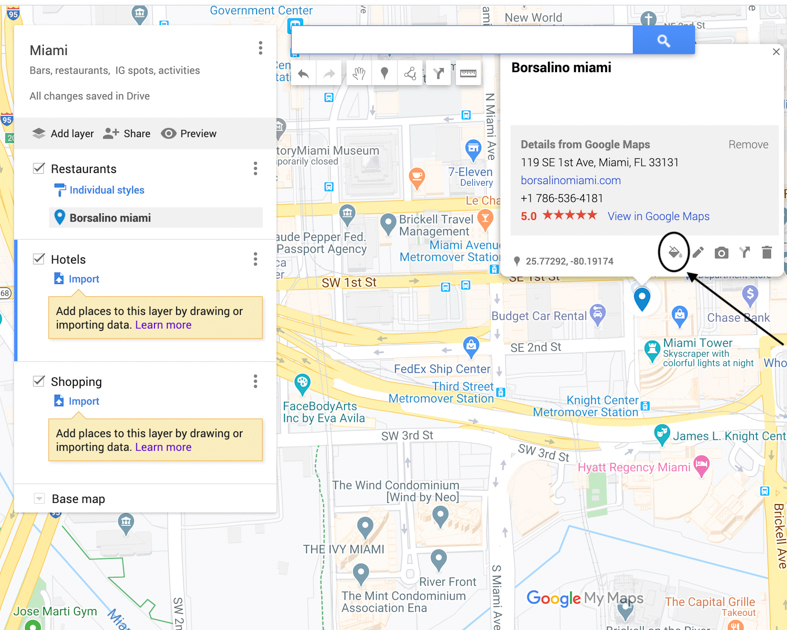This screenshot from Google Maps highlights a detailed view of Borsalino in Miami, FL. Central to the image is the map showing the location of Borsalino at 119 Southeast First Avenue, Miami, FL 33131. To the left, a vertical overlay lists various categories including "Miami," "bars," "restaurants," "IG spots," and "activities," indicating that all changes have been saved in Google Drive. Functions such as adding a layer, sharing, or previewing are also available. 

Checked searches list various categories like "restaurants," "individual styles at Borsalino, Miami," "hotels," "import," and options to "add places to this layer by drawing or importing data," and "learn more." Similarly, under the category "shopping," there are options for "import," "add places to this layer by drawing or importing data," and "learn more." At the bottom, the vertical box includes an option labeled "base map."

In the upper right-hand corner, overlaid on the map, is a square informational box labeled "Borsalino, Miami," providing details such as the official website (borsalinomiami.com), contact number (+1 786-536-4181), and rating (5.05 red stars). A "view in Google Maps" prompt is also included within this box for easy access to more information.